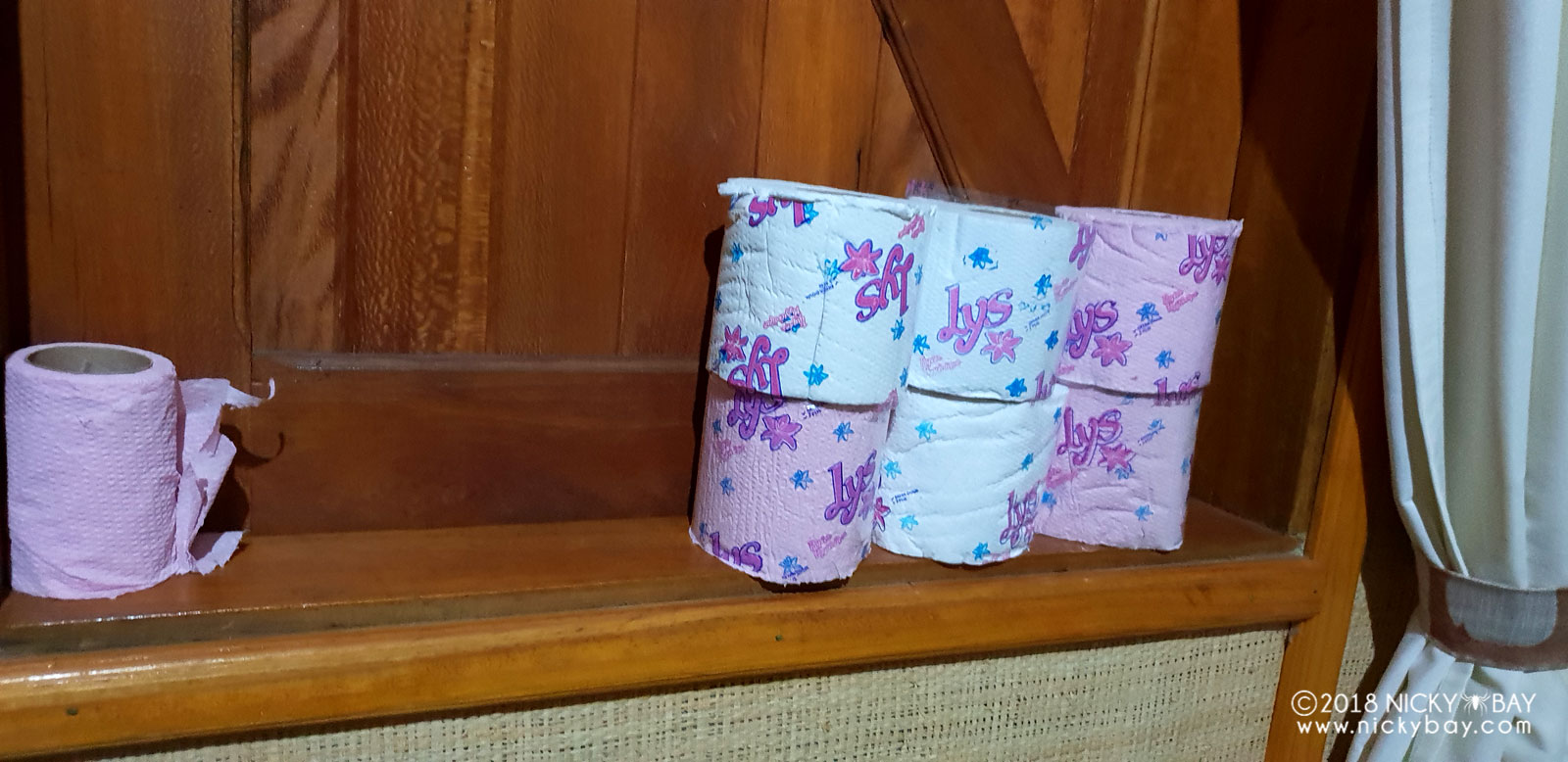This image features a neat arrangement of six rolls of toilet paper, distinctly stacked on an old, reddish-brown wooden shelf. There are three stacks side by side, each two rolls high. The rolls come in white and pink colors, adorned with the letters "J-Y-S" in purple, surrounded by stars and other patterns. Notably, on the left side, there's a partially used and ragged pink roll. To the right, a white curtain tied back with a darker band frames the scene, hinting at a cozy, vintage setting. The shelf, backed by wooden paneling that resembles old speaker fronts or a shuttered window, lends an additional rustic charm to the photograph.